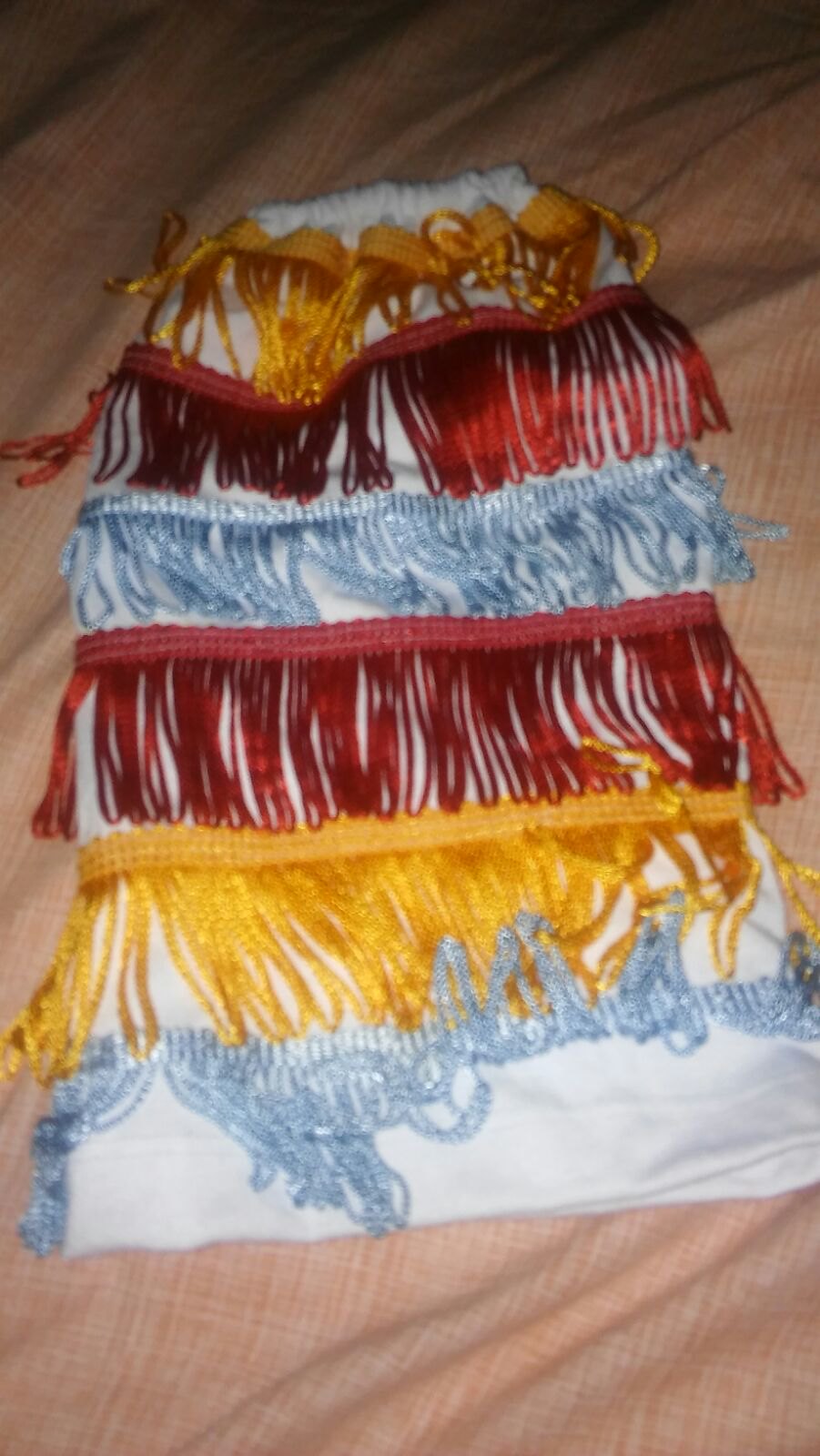This photograph features a detailed image of what likely is a single skirt composed of multiple layers of fringes. The skirt is made from an off-white, sheer, and shiny material with an elastic, gathered top. The various rows of fringe embellishments cascade down the skirt, starting with clusters of red and gold tassels in a bell shape at the top. Beneath this, there are successive layers featuring reddish-brown, silver-green, silver-blue, red, gold, and finally, seafoam-green or seafoam-blue fringes at the bottom.

The skirt lies on a fabric background, possibly a bedspread that is peach or light salmon pink in color and slightly textured with rows of stitched tassels. The background fabric exhibits faint lines and folds, suggesting it isn't smooth and contributes to the visual complexity of the scene. The photograph appears to be taken at night, with noticeable use of flash enhancing the brightness at the bottom of the image while leaving the top relatively dark, indicating uneven lighting and reduced image quality.